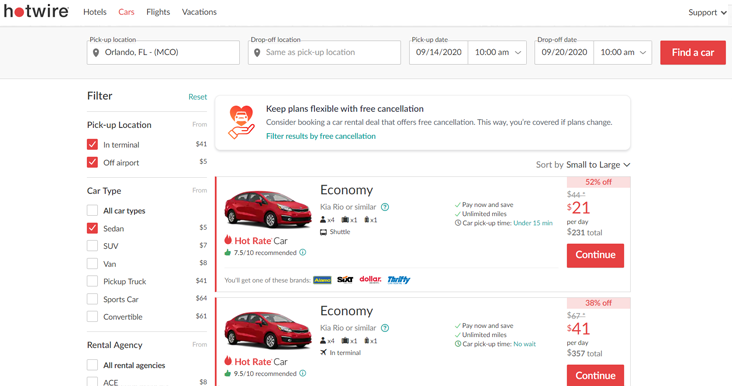This is a detailed screenshot from the Hotwire website showcasing a car rental search. At the top, the input fields indicate that the user has specified Orlando, Florida (MCO) as the rental location, with the option "Same as pick-up location" selected. The rental period is set for September 14, 2020, at 10:00 AM for pick-up, and the car is to be dropped off on September 20, 2020, also at 10:00 AM. 

To the right, there is a prominently featured red button labeled "Find a car." Below this, there are filter options with selections for "In Terminal" and "Off Airport" locations, and the user has chosen a "Sedan" as the car type. 

The search results display options for economy cars, specifically highlighting a "Hot Rate Car," including models such as the Kia Rio or similar. The first option is priced at $21 per day, with a red "Continue" button beneath it, while the second option costs $41 per day, also accompanied by a red "Continue" button.